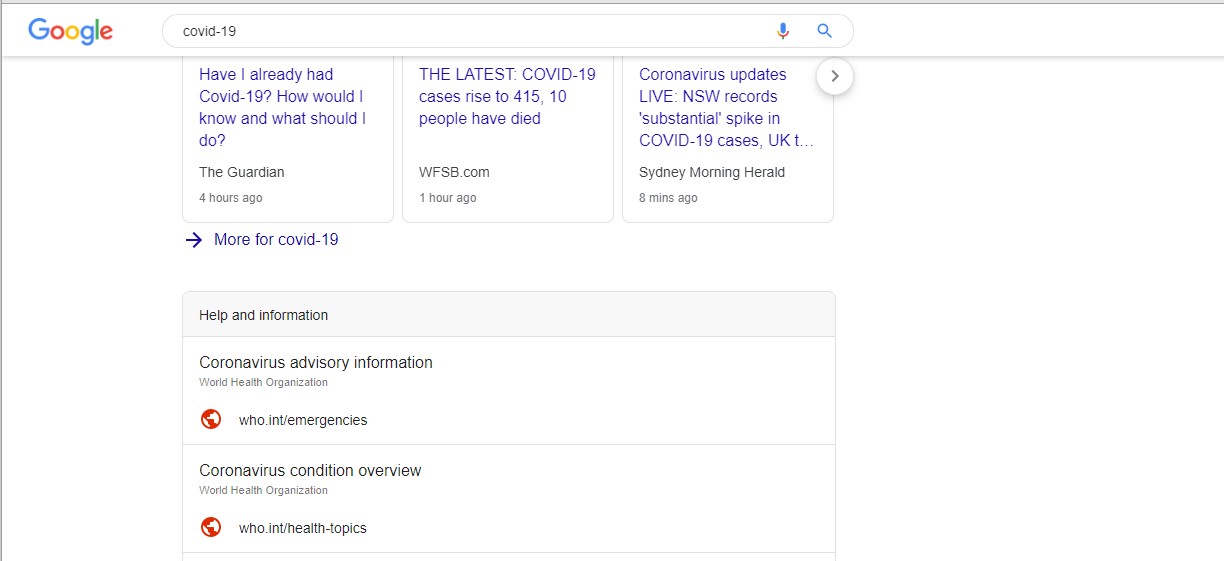The image appears to be a screenshot from Google, featuring a predominantly white background. In the upper left corner, the iconic Google logo is displayed, with a capitalized 'G' in blue, followed by a lowercase 'o' in red, another lowercase 'o' in yellow, a lowercase 'g' in blue, a lowercase 'l' in green, and finally a lowercase 'e' in red. To the right of the logo, there is a search bar where the term "COVID-19" has been typed. Positioned at the far right of the search bar are a microphone icon and a magnifying glass icon, indicating options for voice search and standard search, respectively.

Below the search bar, there are three primary result blocks displayed as small squares:
1. The first block on the left features the headline: "Have I already had COVID-19? How would I know, and what should I do?" This result is from 'The Guardian' and was published four hours ago.
2. The middle block reports: "The latest COVID-19 cases rise to 415, 10 people have died," sourced from 'WFSB.com' one hour ago.
3. The third block on the right headlines: "Coronavirus updates live: NSW records substantial spike in COVID-19 cases," attributed to 'Sydney Morning Herald' from eight minutes ago.

Below these blocks, there is an arrow pointing to the right with the label “More for COVID-19,” suggesting additional information can be found by following the link.

Further down, a gray heading reads "Help and Information," beneath which are two rectangular sections:
1. The first rectangle is labeled "Coronavirus Advisory Information."
2. The second rectangle is titled "Coronavirus Condition Overview."

This highly detailed screenshot captures a snapshot of real-time COVID-19 updates and informational resources provided by Google.